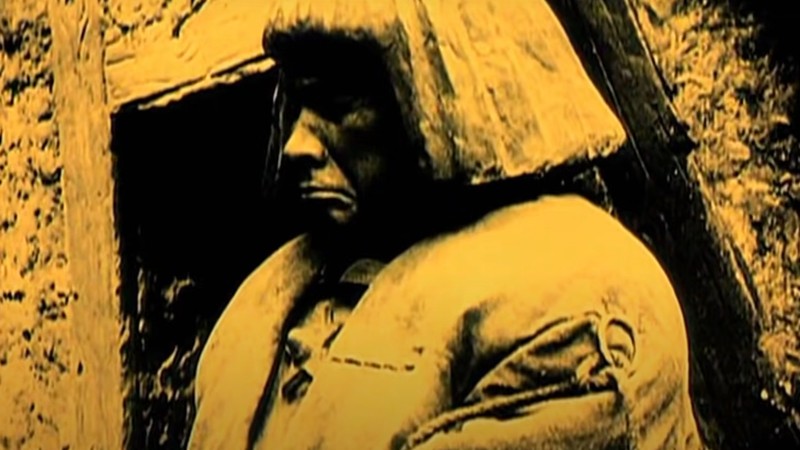The image depicts a sepia-toned, early photograph with a yellowish tint, featuring a Native American figure seated in front of a doorway. The subject has straight hair or possibly a head covering that falls just above the shoulders, and is wearing a heavy jacket adorned with military-like rope detailing on the shoulders. Notably, he appears to have a sheriff's star on his chest, indicating he might be a deputized sheriff. The doorway he is sitting before is framed with timber, and the surrounding building material appears to be a combination of stone, mud, and thatch. Despite the black and white nature of the photograph, the yellow tint emphasizes the period's antiquity while obscuring some finer details, such as the exact texture and material of the building and the individual’s facial features.